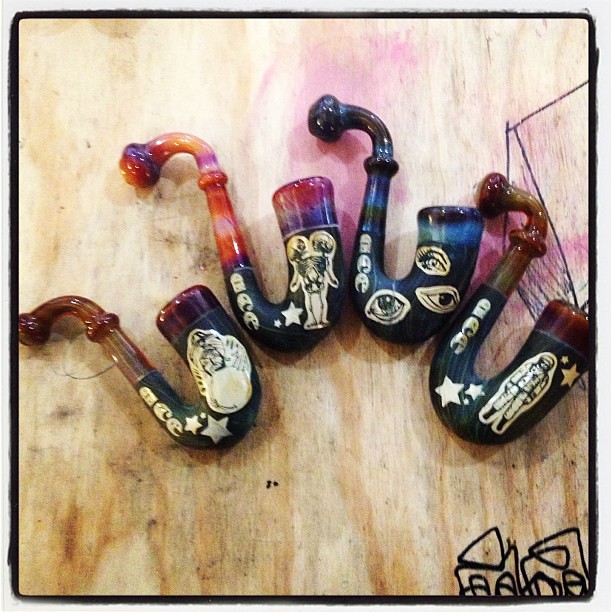The image features four intricately designed glass pipes, each distinctly colorful and laid out on a rustic, light brown barn wood table. The wooden surface provides a contrasting backdrop that highlights the vibrant hues of the pipes. Each glass pipe showcases a black wrapping adorned with white illustrations: one displays an astronaut amidst stars, another features an array of eyes, the third presents a two-headed skeleton, and the fourth, while partially obscured, appears to have celestial imagery.

From left to right, the pipes are as follows: the first pipe has a dark blue body transitioning into a purple top. Its base is adorned with a wrap depicting eyes. The second pipe is richly multicolored, sporting shades of orange, pink, yellow, and red, with a bowl head in purple and pink, wrapped with imprints of an alien. The third pipe, primarily blue with black highlights, also includes eyeball illustrations. The final pipe possesses a brown and green body with a wrap that has the astronaut imagery.

Adding to the depth of the scene, a signature sketched in black ink is discernible at the bottom right corner of the image, though the exact wording remains unclear. Encasing the entire image is a subtle black border followed by a slim margin of light gray.